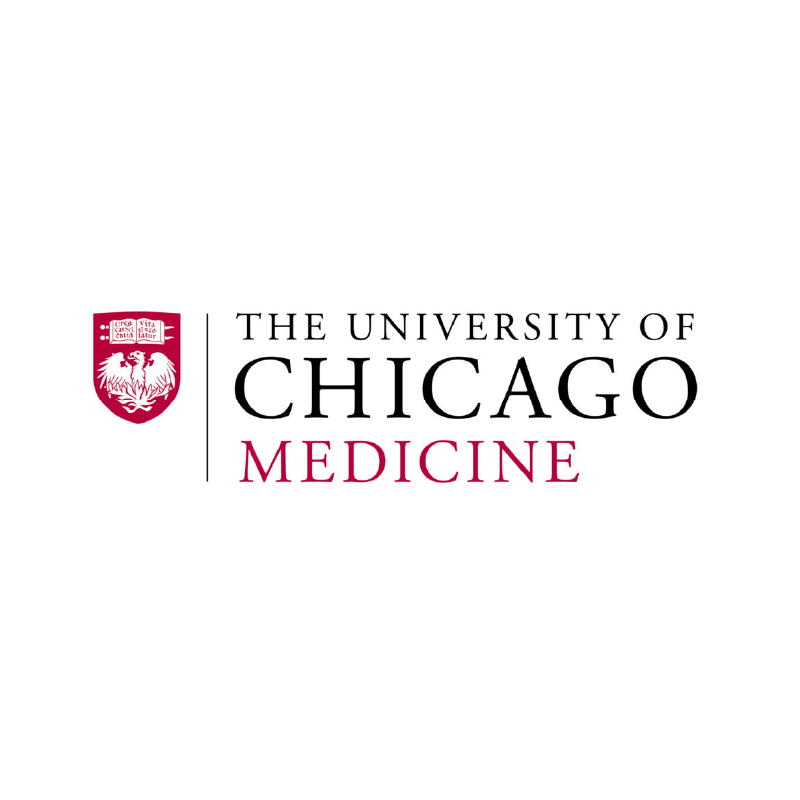The image features the logo of the University of Chicago Medicine prominently centered within the frame. The overall dimensions of the image include approximately 40% blank space both above and below the logo, which occupies around 20% of the image height.

On the left side of the logo, there is a distinctive crest in red. This crest features a white eagle, or possibly a phoenix, with outstretched wings. Flames lick upwards from below the bird, suggesting a phoenix rather than an eagle. Above the bird, there is an open book with visible letters including "C," "V," and partial words like "veto" and "eco" on three lines of text, indicating a Latin motto. The pages of the book also display two skewers or swords crossing through the center, one with round ball-like ends.

The bird’s head is turned to the left, with what appears to be either a tongue or flames emerging from its mouth. A thin black horizontal line separates this crest from the accompanying text.

To the right of the crest, the text of the logo is in capital letters. First, 'The University of' is written in black, smaller font. Directly below, in a larger font size also in black, is 'CHICAGO,' stretching the full width of the text block above. Finally, the word 'MEDICINE' is written in red, slightly larger than 'The University of' text but smaller than 'CHICAGO.' The word 'MEDICINE' spans about three-quarters of the width of the black text. All the text elements are in uppercase letters.